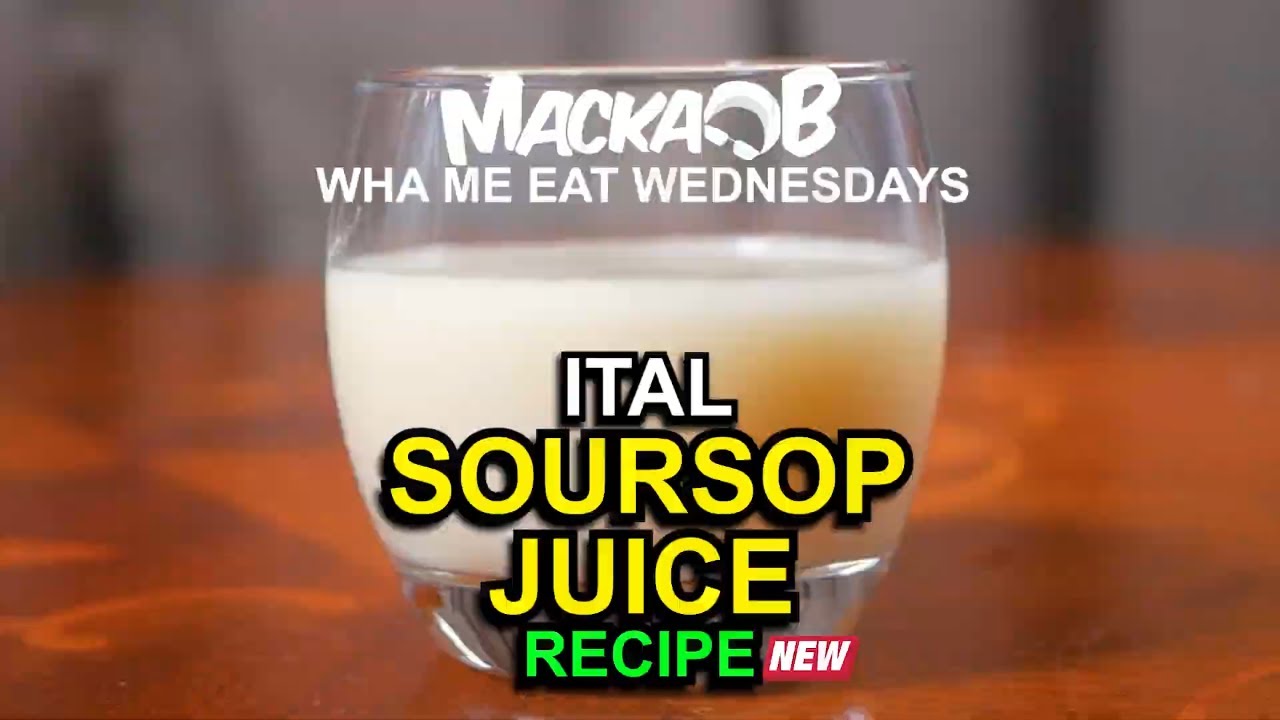The image shows a clear glass filled about three-quarters of the way with a whitish liquid, which might also have some brown hues. The glass is positioned on an orangey wood-colored table that is blurred in the background, suggesting an indoor setting. Superimposed over the glass, there is text that reads "MACAOB Wah Me Eat Wednesdays ITAL Soursop Juice Recipe New." The word "MACAOB" is written in white at the top, followed by "Wah Me Eat Wednesdays," also in white. "ITAL" is prominently displayed in white, while "Soursop Juice" is in yellow with a black outline, and "Recipe" is in green with a black outline. The word "New" appears in white letters on a red banner-like background. The details hint at a promotional image, possibly an advertisement for soursop juice, under the brand "MACAOB."